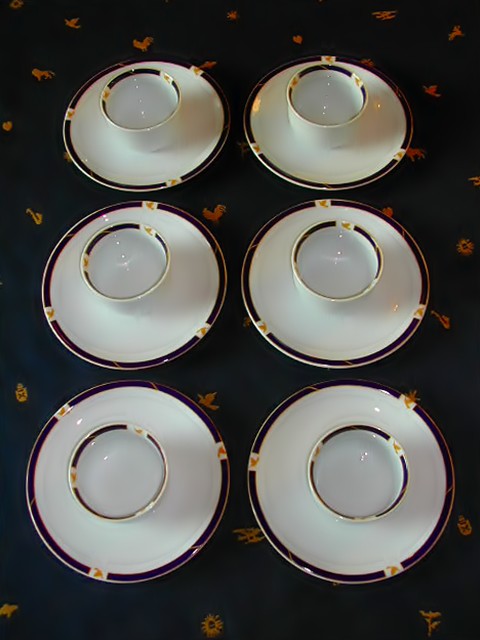This image features six white teacups and their matching saucers, each adorned with a distinct brown edging. The cups and saucers showcase a repeating pattern featuring three small designs on both the cup and saucer edges, likely depicting abstract forms like leaves or birds. These are neatly arranged in two rows of three, aligned side by side, suggesting a two-by-three layout.

The set is displayed on a background that appears to be a dark fabric, potentially a navy blue napkin with intricate, tiny designs, including flowers, leaves, birds, and other indistinct shapes like a saxophone and a helicopter. This layout provides an overhead view, emphasizing both the symmetry and the decorative details of the teacups and saucers. Despite the lack of information on the manufacturer or specific purpose, the cups capture reflections from the light source, contributing to their visual appeal against the detailed backdrop.